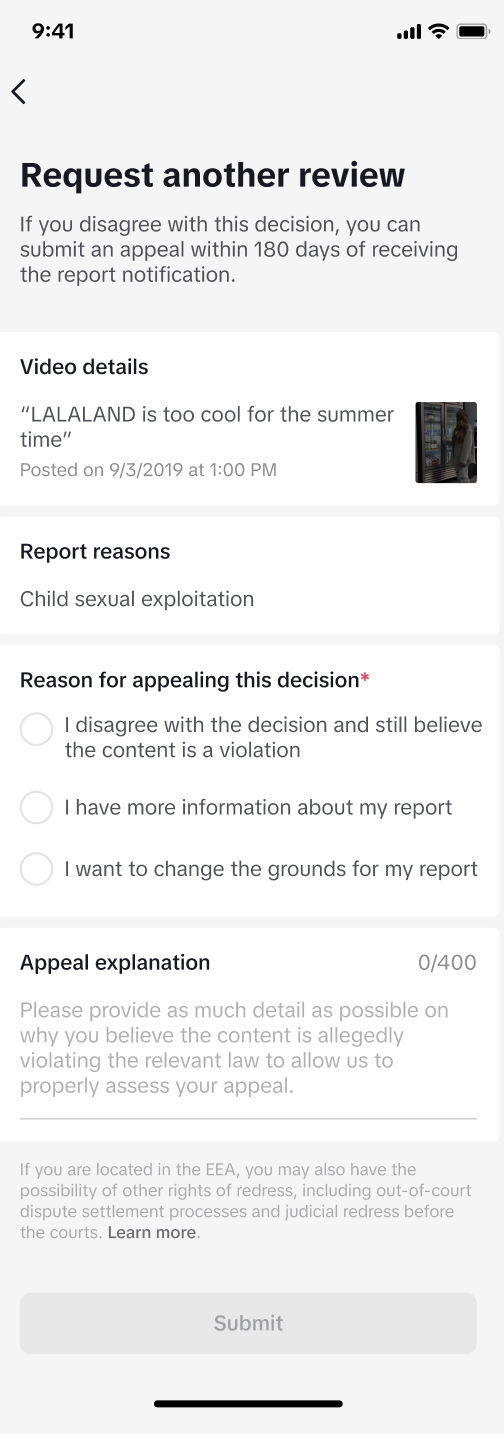A detailed view of an appeal form on a video sharing platform is displayed. The form is designed for users to request another review of a reported video. It offers a clear explanation that, if a user disagrees with the initial decision not to remove the video, they can submit an appeal within 180 days of receiving the report notification. The video in question, titled "La La Land is Too Cool for the Summer Time," was posted on September 3, 2019, at 1 PM and was reported for reasons related to Child Sexual Exploitation. 

The form includes options for the user to specify their reason for appealing the decision. These options include:
1. Agreeing with the decision but still believing the content is a violation.
2. Disagreeing with the decision.
3. Providing additional information about their report.
4. Changing the grounds for their report.

Furthermore, there is a section labeled "Appeal Explanation," where users are encouraged to provide as much detail as possible to explain why they believe the content violates relevant law. This section aims to gather extensive information to assist in the re-evaluation of the reported content. It is implied that the user believes the video in question should not have been allowed and is taking steps to bring this to the attention of the platform’s moderators.